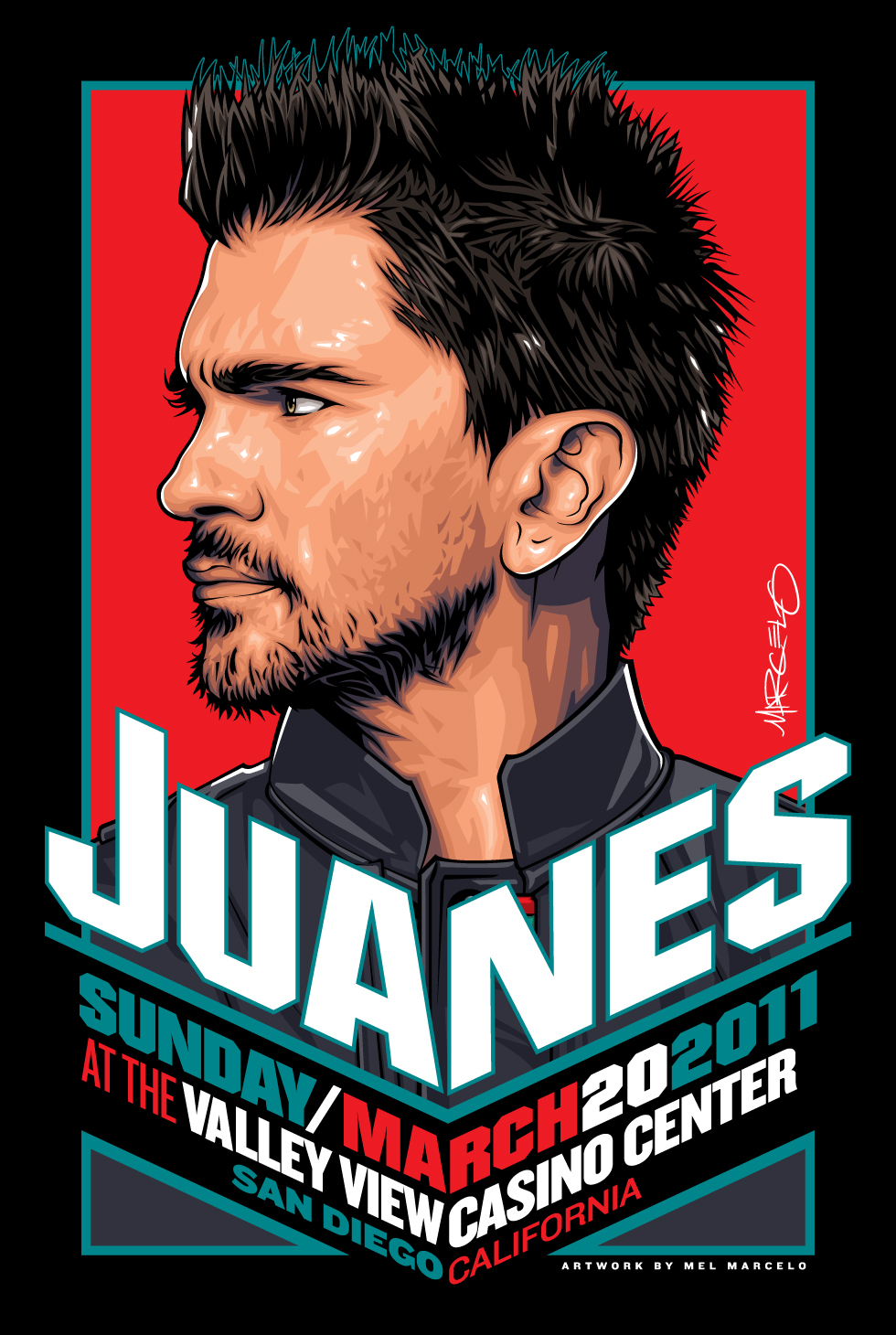This vibrant poster advertisement features an artistic rendering of a young man named Juanes, scheduled to perform on Sunday, March 20th, 2011, at the Valley View Casino Center in San Diego, California. The captivating artwork showcases Juanes in a side view, with his short, spiky brown hair, subtle mustache, and goatee, all against a red background. He is depicted sporting a high-collared jacket. The poster's color palette predominantly uses the shades of the Mexican flag—green, red, and white—along with accents of dark turquoise. At the bottom right corner, it credits the artwork to Mel Marcello, adding a touch of artistic authenticity to the already striking visual.